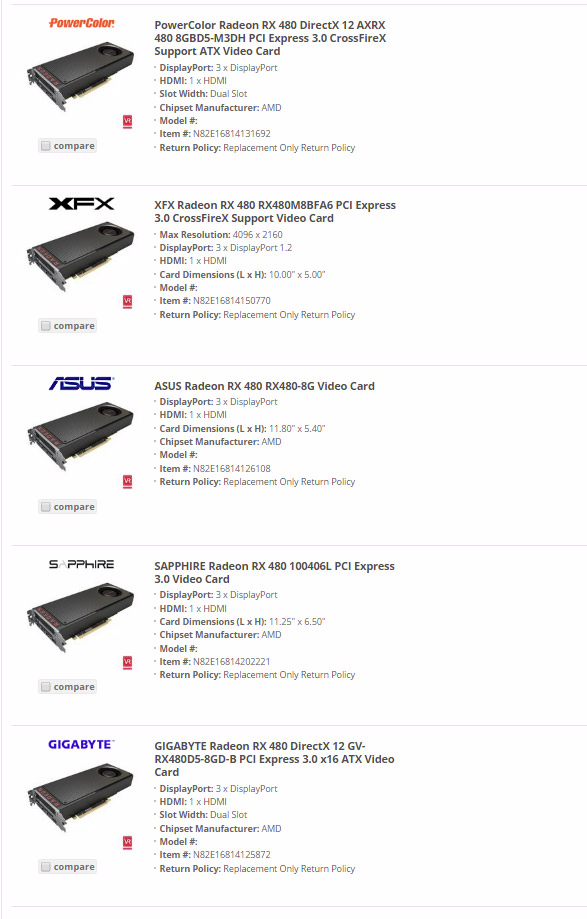This image displays a comparison of various graphics cards, highlighting their key specifications and features. The focus is on multiple Radeon RX 480 models from different manufacturers, showcasing their compatibility with DirectX 12 and PCI Express 3.0, as well as their support for Crossfire X.

1. **PowerColor Radeon RX 480**: 
   - **Model**: AX-RX-480-8GBD5-M3DH
   - **Memory**: 8GB DDR5
   - **Video Outputs**: 3x DisplayPort, 1x HDMI
   - **Form Factor**: Dual-slot ATX
   - **Chipset Manufacturer**: AMD
   - **Item Number**: N82E16814131669
   - **Return Policy**: Replacement only

2. **XFX Radeon RX 480**: 
   - Detailed specifications are not fully provided, but it is highlighted as the second model in the comparison.

3. **Sapphire Radeon RX 480**: 
   - **Model**: 100406L
   - Detailed specifications are not expanded upon in the provided description.

4. **Gigabyte Radeon RX 480**: 
   - **Model**: GV-RX480D5-8GB
   - **Memory**: 8GB
   - **Compatibility**: DirectX 12

The comparison illustrates the variety of Radeon RX 480 graphics cards available, emphasizing their capacity for high performance in gaming and graphical applications, facilitated by their support for dual-slot configurations, ample memory, and robust output options.